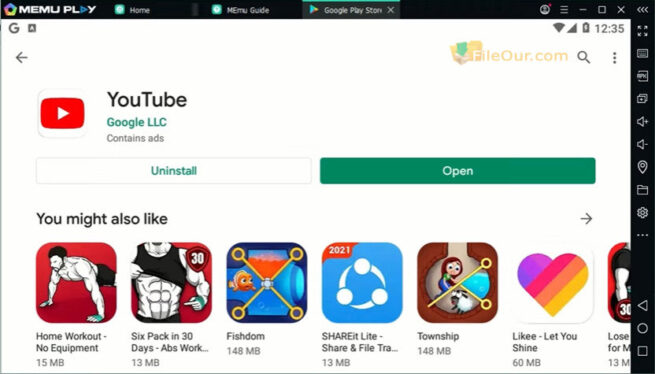This image is a screenshot taken from a YouTube video displaying an old interface on a computer or laptop screen. The screenshot includes a black banner running across the top and down the right side. In the top-left corner of the banner, there is a colorful icon next to the text "Mimu Play." To the right, there are buttons for "Home," "Menu Guide," and the "Google Play Store." Various computer icons line the right edge of the screen.

The main section of the screenshot focuses on the YouTube app details in the Google Play Store. A red play button is displayed prominently with the text "YouTube" beside it, followed by "Google LLC" and "Contains ads." Below this, there is a white banner with a green "Uninstall" button and a green banner with a white "Open" button.

Further down, a section titled "You might also like" showcases six app suggestions. The first app is "Home Workout - No Equipment," followed by "Six Pack in 30 Days." The third suggestion is a game called "Fishdom." The fourth app is "SHAREit Lite: File Sharing & Transfer." The fifth is a game titled "Township," while the sixth app features a heart icon and the text "Likee - Let You Shine." The final, partially visible, app seems to be related to weight loss, depicted by an icon of a person with a dumbbell.